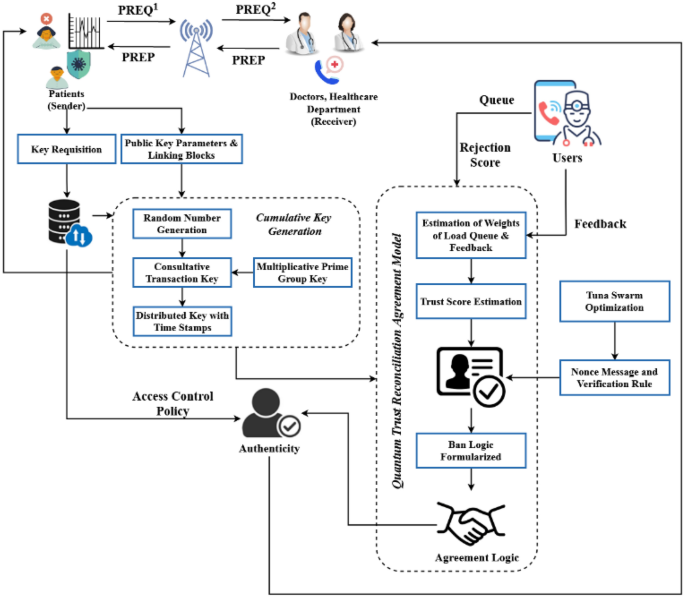The diagram illustrates a complex system of medical information flow, depicting the relationships and processes among various healthcare entities and personnel. Central to the diagram are head-and-shoulders images of a female and a male healthcare professional, possibly doctors or nurses, each with a stethoscope around their necks. These figures are identified as part of the "Health Care Department" and are labeled as "Receivers." 

Arrows and connecting lines criss-cross the diagram, linking a series of blue blocks and labeled boxes that represent various stages and elements of information transfer. Key labels include "P-R-E-Q," "P-R-E-Q-2," and terms such as "patient," "sender," "queue registrations," "public key parameters," "trust score estimation," "multiplicative prime group key," "access control policy," and "authenticity." Specific pathways are highlighted, including a line from "queue" to "rejection store" and from the healthcare professionals to "user feedback."

Additionally, the diagram seems to emphasize reducing the steps a patient or user must take to send or retrieve information, suggesting an optimized communication network. The overall arrangement, with elements like "doctor with his telephone" and "nurse" image placements, outlines how information travels through this interconnected system, focusing on efficient and secure healthcare communication processes.